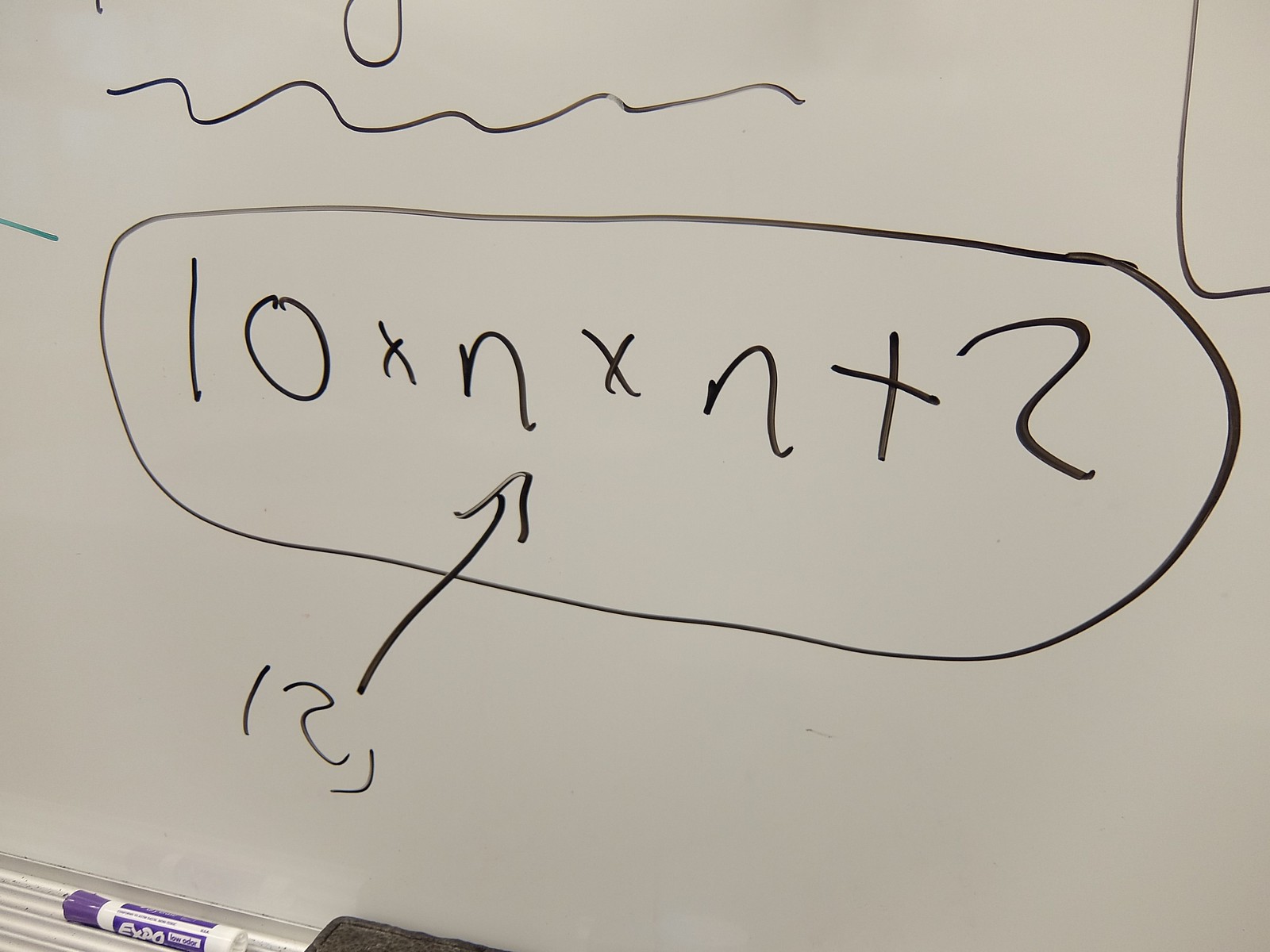This is a detailed photo of a math equation, written on a whiteboard in black marker. The equation reads "10xn * n + ?", enclosed in an oval. An arrow points to the equation, and beneath the arrow is the notation "12" or "( ) to ( )". Above the circled equation, there's a squiggly line with a 'U' pattern, accompanied by random lines and dashes scattered around. An Expo marker and the top edge of the silver ledge are visible at the bottom of the whiteboard.